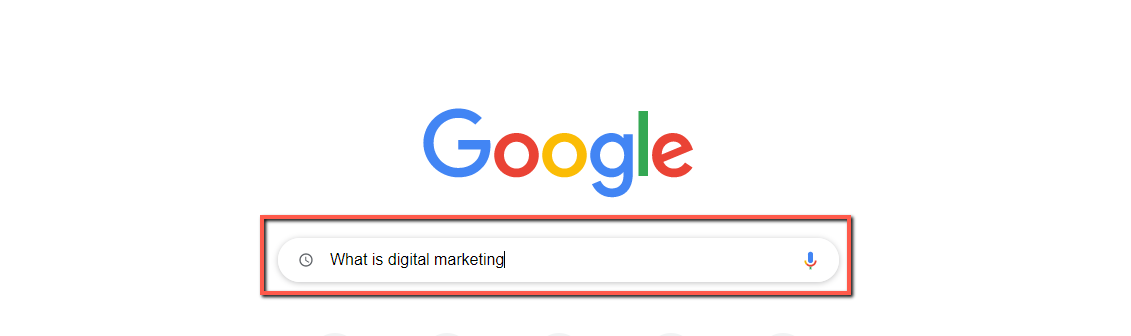The image showcases the iconic Google homepage, characterized by its simple and clean design. Dominating the page is the recognizable Google logo, which features the company's signature colors: blue, green, yellow, and red, all set against a plain white background.

Centering the page, directly beneath the logo, is a search bar encapsulated within a box. The box features a subtle light blue border, though red appears to be the most dominant color around it. Within this, the search bar itself sits prominently in a long, rounded rectangle shape. The background around the search bar remains white, maintaining the minimalist aesthetic.

Inside the search bar, the placeholder text "What is digital marketing?" is visible, with the text cursor situated right after the letter 'G.' To the left of this search query, there is a small, rounded search icon that signifies the search function. At the far right of the search bar, there is a microphone icon, which allows users to perform voice searches by speaking instead of typing.

The overall composition conveys the straightforward and user-friendly design of the Google search interface, emphasizing its functionality and easily recognizable elements.